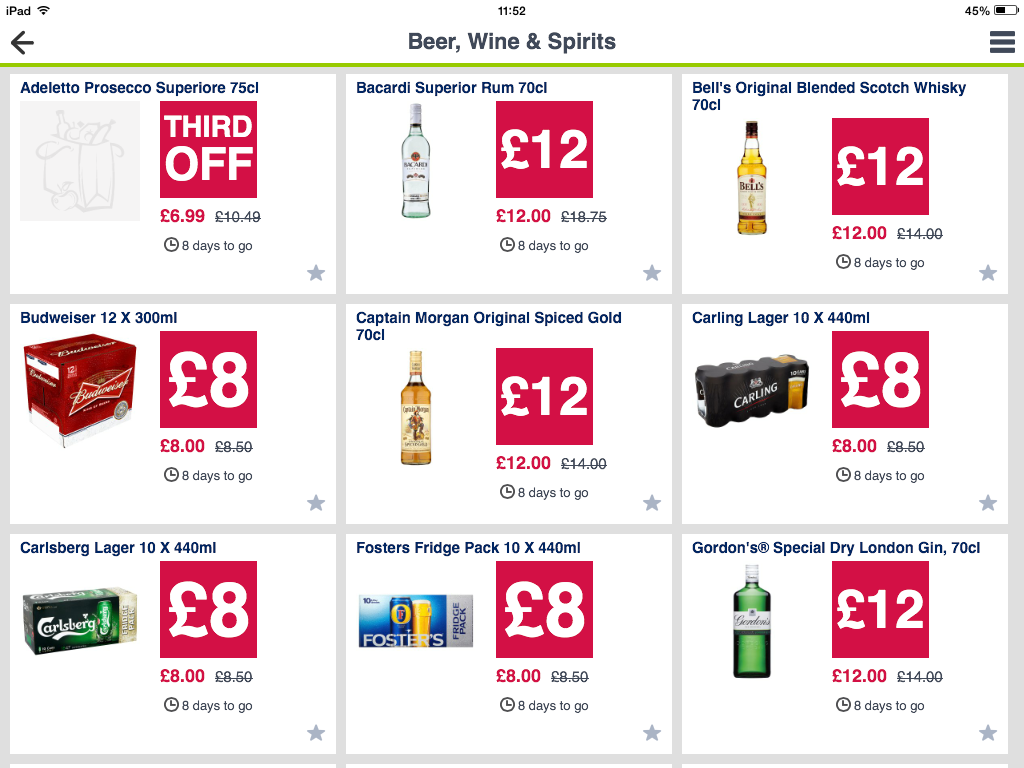**Detailed Image Description:**

The image is a screenshot taken on an iPad, showcasing a selection of online coupons for various alcoholic beverages. The iPad interface is visible, with the "iPad" label in the top-left corner, a Wi-Fi signal icon in the top-right, and a battery icon indicating 45% charge. The time displayed at the center of the screen is 11:52.

Below this information, the screenshot features a section with the heading "Beer, Wine, and Spirits" in black text, underlined by a very thin green line. Adjacent to this heading, on the left side, there is a back arrow icon, and on the right, there are three horizontal bars representing a menu.

The main content displays a 3x3 grid with a gray background, comprising nine rectangular coupon items. Each coupon has a white background, resembling a piece of landscape-oriented computer paper. The items are arranged from left to right and top to bottom as follows:

1. **Adaletto Prosecco Superiori 75 cl** - A 30% discount coupon.
2. **Bacardi Superior 70 cl** - Priced at £12.
3. **Bell's Original Blended Scotch Whisky 70 cl** - Priced at £12.
4. **Budweiser 12 x 300 ml** - Priced at £8.
5. **Captain Morgan Original Spice Gold 70 cl** - Priced at £12.
6. **Carling Lager 10 x 440 ml** - Priced at £8.
7. **Carlsberg Lager 10 x 440 ml** - Priced at £8.
8. **Foster's Fridgepack 10 x 440 ml** - Priced at £8.
9. **Gordon's Special Dry Lemon Gin 70 cl** - Priced at £12.

Each coupon features the respective product image, description, size, and price or discount information, providing a comprehensive overview of the available deals on alcoholic beverages.